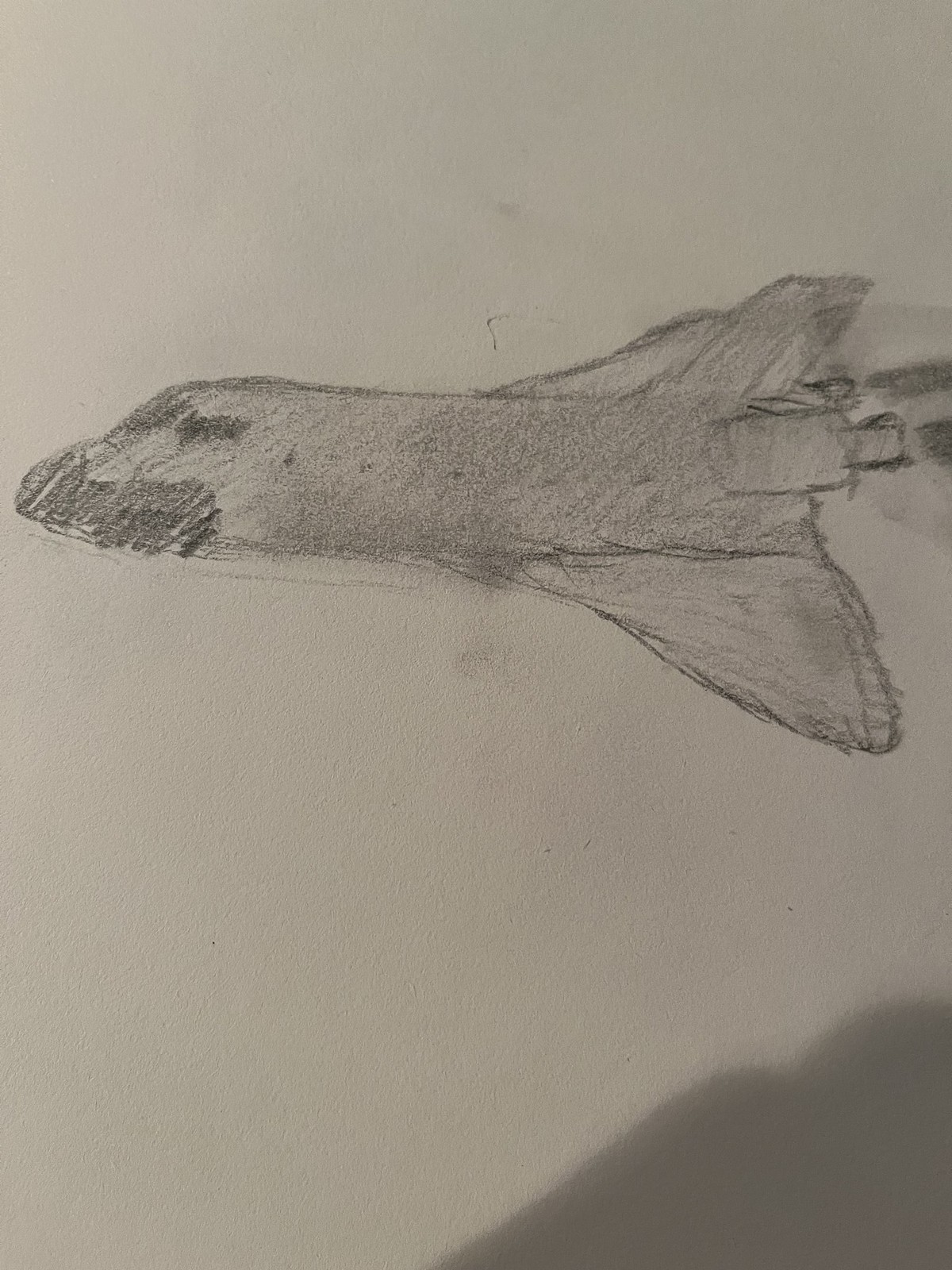This pencil drawing on a white piece of paper features a side view of an airplane, which may also be interpreted as a space shuttle, flying to the left. The artist has given the airplane a whimsical touch, making the front of the aircraft resemble a face: the windows appear as eyes, and a darker shaded area suggests the presence of a mouth. Despite its fanciful elements, the airplane is identifiable by key features such as its wings and tail. At the rear, a stream of gas or smoke is depicted, indicating motion. While the drawing showcases moderate shading and attention to detail, it remains relatively simple and straightforward in its execution.